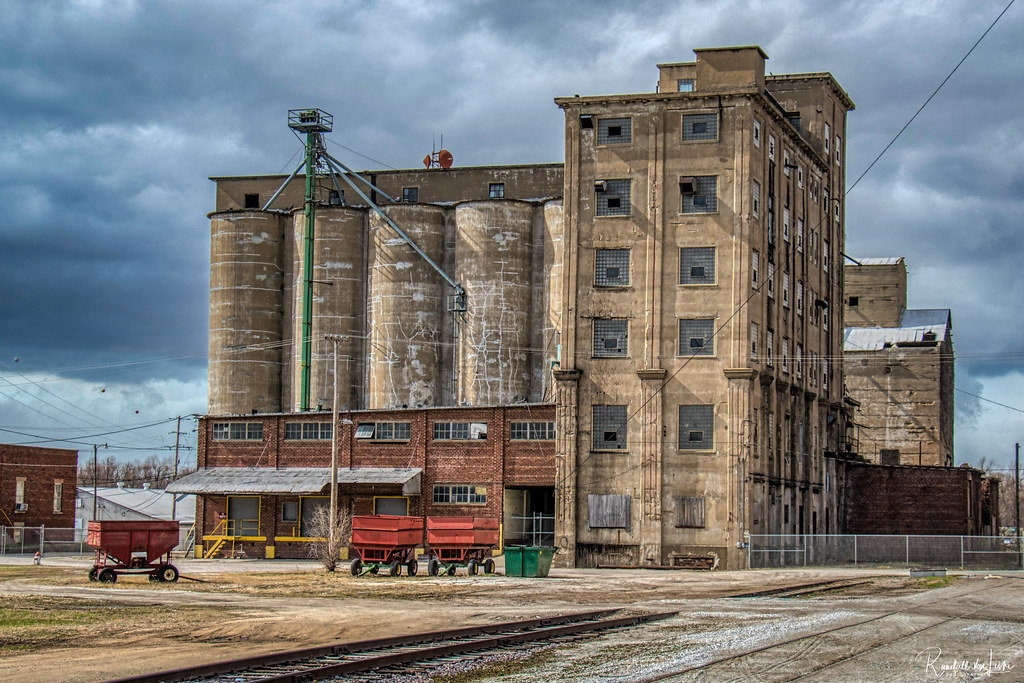This color photograph depicts a large, multi-story industrial building, likely a grain facility. The building, constructed of brick, stands six stories tall and features windows with small glass grids, each equipped with ventilation. Attached to the building are five cylindrical silos, as tall as the building itself, connected by pipes and a tall green auger. Surrounding the facility is a chain-link fence, and adjacent to the building are brown structures, including a smaller dark brown two-story building. There are no vehicles or people present, suggesting it may be vacated.

In the foreground, three orange carts designed for material transport are visible, along with a green garbage can. The ground is covered in gravel and dirt, interspersed with railroad tracks, and patches of grass. The shipping docks at the building's front or side have been painted yellow, and feature orange metal iron docking for trailer truck loading. The overcast sky is dominated by heavy gray clouds, adding to the desolate atmosphere. The photograph also contains a signature with a prominent 'R' in the bottom right corner, though the rest of the name is illegible. Visible colors in the image include various shades of brown, green, orange, gray, and white.